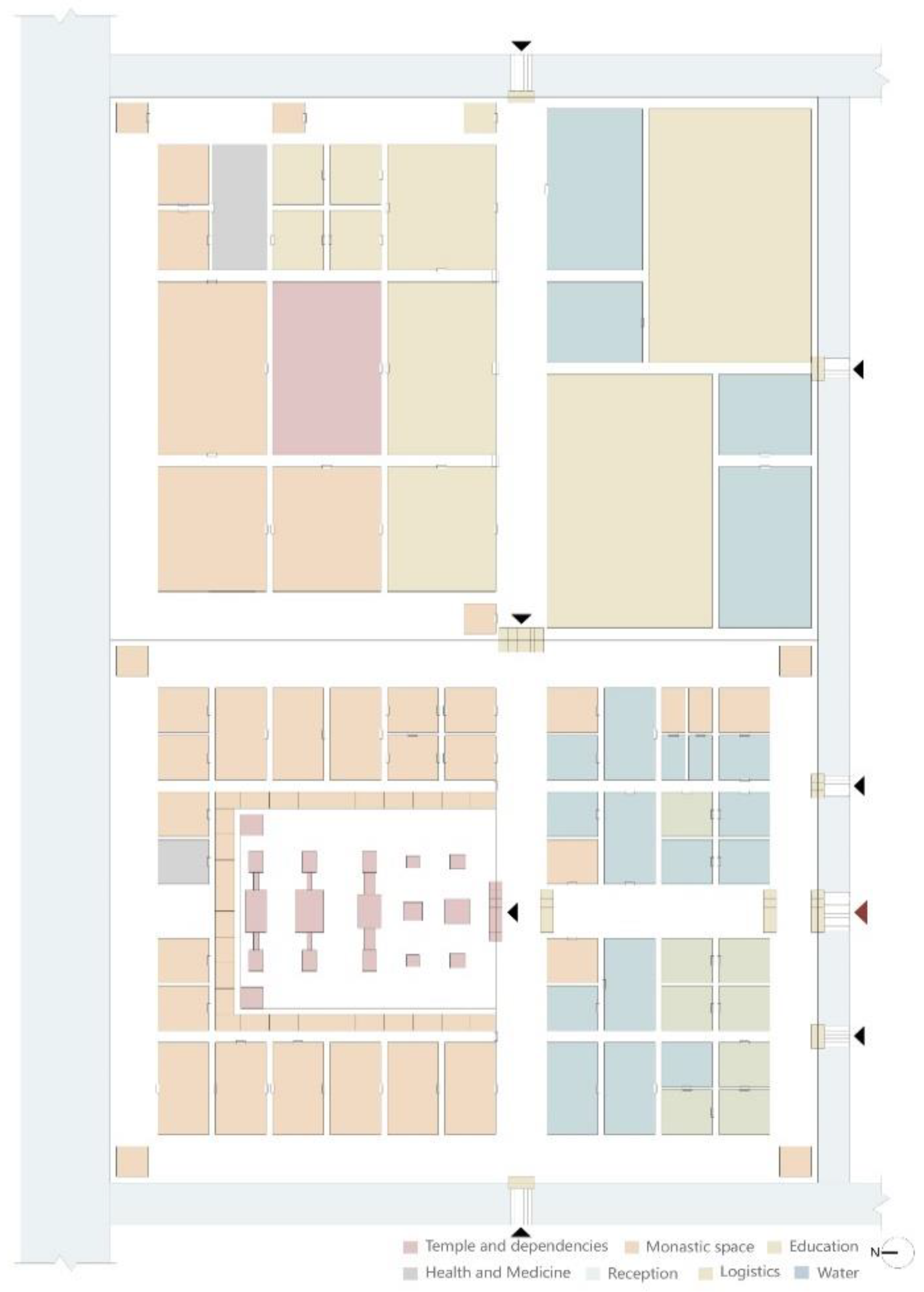This image appears to be a detailed, computer-generated blueprint or floor plan of a building, rendered exclusively as an illustration with no photographic elements. The layout reveals a large rectangular structure divided into various smaller and larger colored rectangles, each representing different sections of the building. These sections include labels such as Temple and Dependencies, Monastic Space, Education, Health and Medicine, Reception, Logistics, and Water, as indicated by a key located at the bottom of the image. Multiple black arrows are drawn to indicate entrances and exits throughout the building. The floor plan features a range of colors including blue, beige, and purple, with some white spaces interspersed. The specific name of the building is not provided, and there are no people or animals depicted in this meticulous architectural illustration.